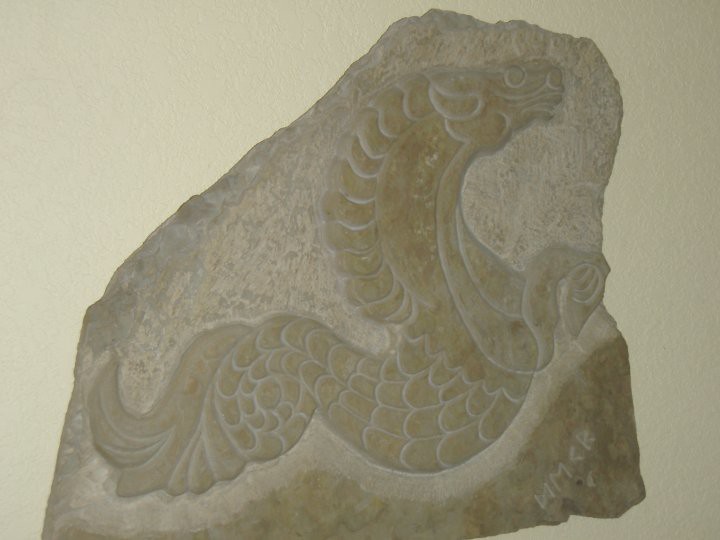This color photograph depicts a detailed carving on a trapezoidal grey stone, which is positioned against a beige or off-white wall. The central figure etched into the stone is an imaginative, hybrid creature combining elements of a horse and a fish. The creature features the head, mane, and front hooves of a horse, along with a body adorned with scales that tapers into a pointed tail, resembling that of a fish or snake. The carving exhibits intricate details, such as the long neck and the oddly angled hooves of the creature. Alongside the figure's detailed contours, the stone surface transitions from a smooth, carved section around the creature to a rough, untouched section at the bottom. In the bottom right corner of the stone, the letters "MMCK" are clearly engraved. This unique amalgamation of different animal features, masterfully carved into the stone, captures a blend of natural and mythical elements.